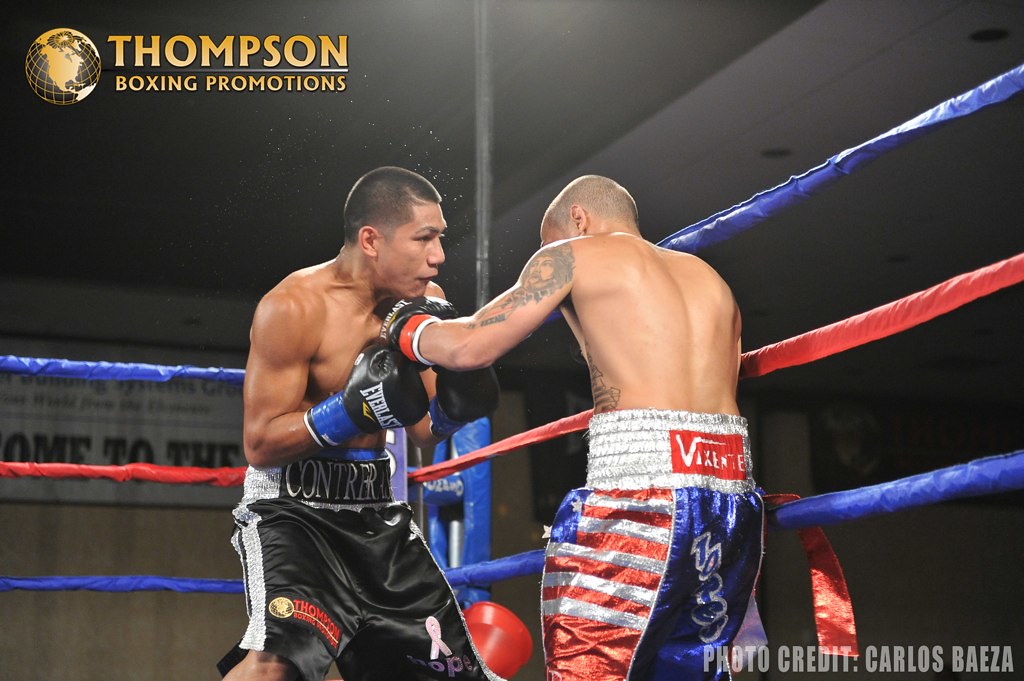In this vibrant promotional image from Thompson Boxing Promotions, captured by photographer Carlos Baeza, two young boxers are locked in intense action within a vividly colored ring. The ring features three ropes: the upper and lower ropes are blue, while the middle rope is green. In the upper left corner of the image, there's a golden globe logo with the text "Thompson Boxing Promotions." The boxer on the left, identified by his American flag-themed shorts in red, white, and blue, is attempting to block a left hook from his opponent. This opponent, positioned on the right, has tattoos on his arms and sides and is wearing black shorts featuring various symbols, including a pink breast cancer ribbon on his left leg and gray lettering. This encounter takes place near the corner of the ring, behind which an advertising sign partially reads, "come to the." The dynamic composition captures the moment of impact as the boxer on the right delivers a punch to his opponent's chin, emphasizing the raw intensity and athleticism of the match.